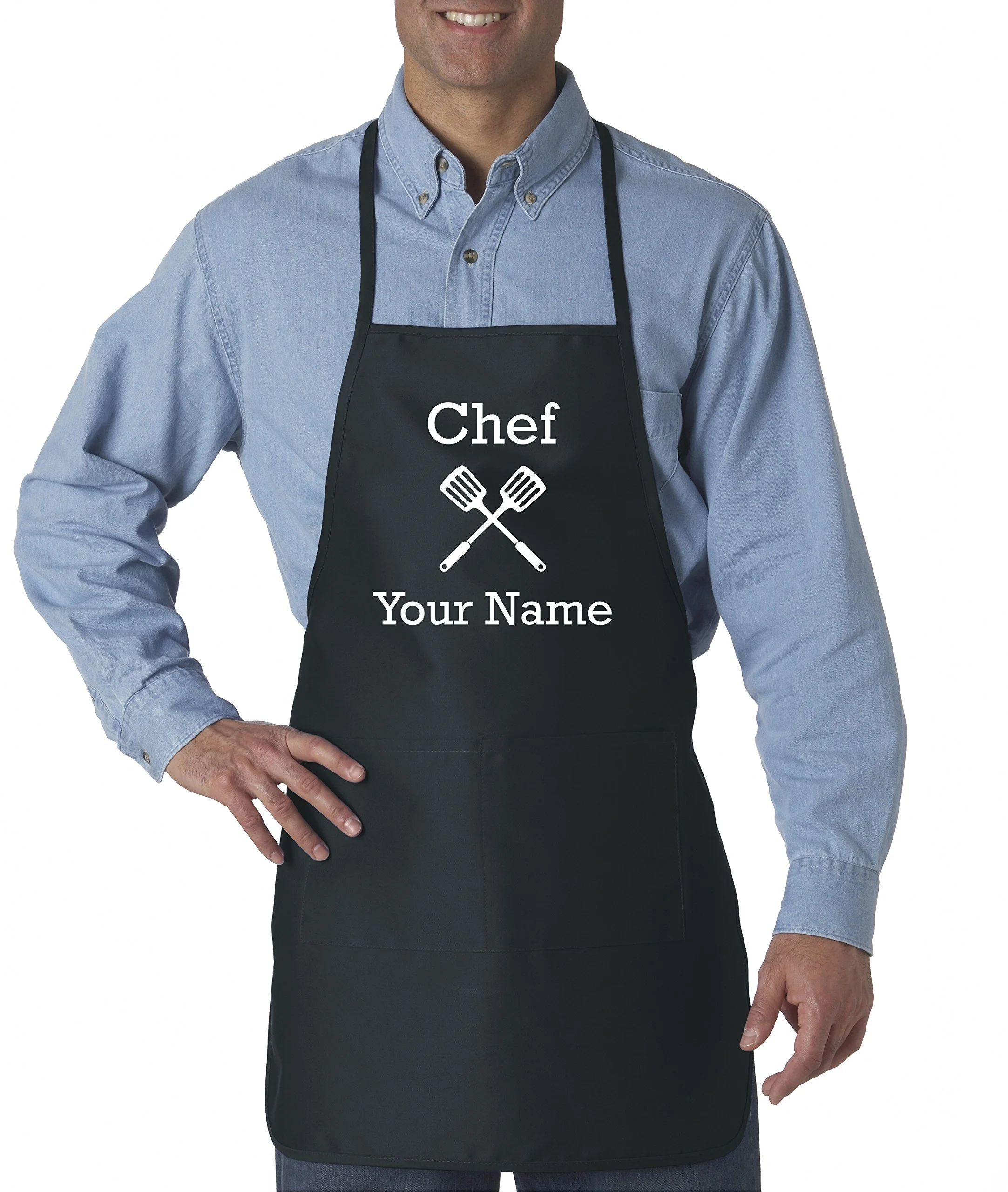The image depicts a white man, clean-shaven, standing confidently with his right hand on his hip. He is posed against a stark white background that emphasizes the central focus of the photo—him and the black apron he is wearing. The man is dressed in a long-sleeve, blue denim button-up shirt, with the top button casually left open, paired with blue jeans. Over his attire, he sports a black apron that is customizable, prominently featuring the words "Chef Your Name" in white lettering across the front, along with two crossed spatulas above the text. This apron is clearly designed for personalization. The man is smiling, showcasing his white teeth, which adds a welcoming and friendly touch to the image. Although the photo is framed from the middle of his thighs to just above his mouth, the professional presentation and realistic customization depiction make it clear that this is likely a stock image intended for an online marketplace, such as Amazon, to advertise a customizable chef apron.